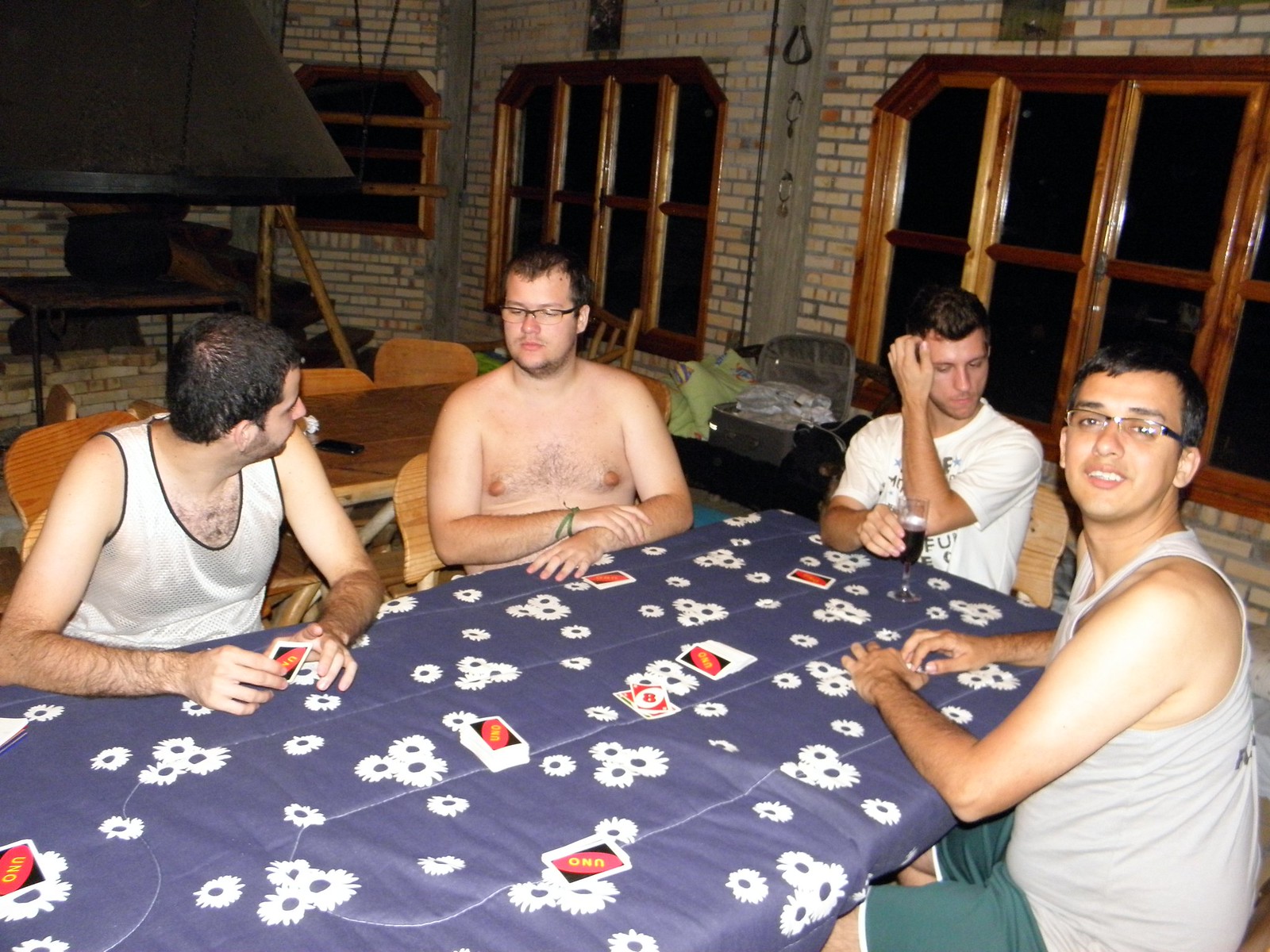In the photo, four men are gathered around a blue tablecloth adorned with white sunflower patterns, playing a game of Uno indoors. The man on the far right is wearing a grey tank top and green shorts, along with glasses, and is looking directly at the camera. To his left, a man in a white t-shirt holding a half-filled wine glass in his right hand is scratching his head with his left hand, looking downward. Further to the left, a shirtless man with glasses is seated, his eyes closed and head turned slightly to the left. The leftmost man, dressed in a white tank top, is focused on the shirtless man next to him while holding a set of Uno cards. The background features beige brick walls, wooden windows, additional tables, open suitcases, and pillows, suggesting a homey, casual setting.